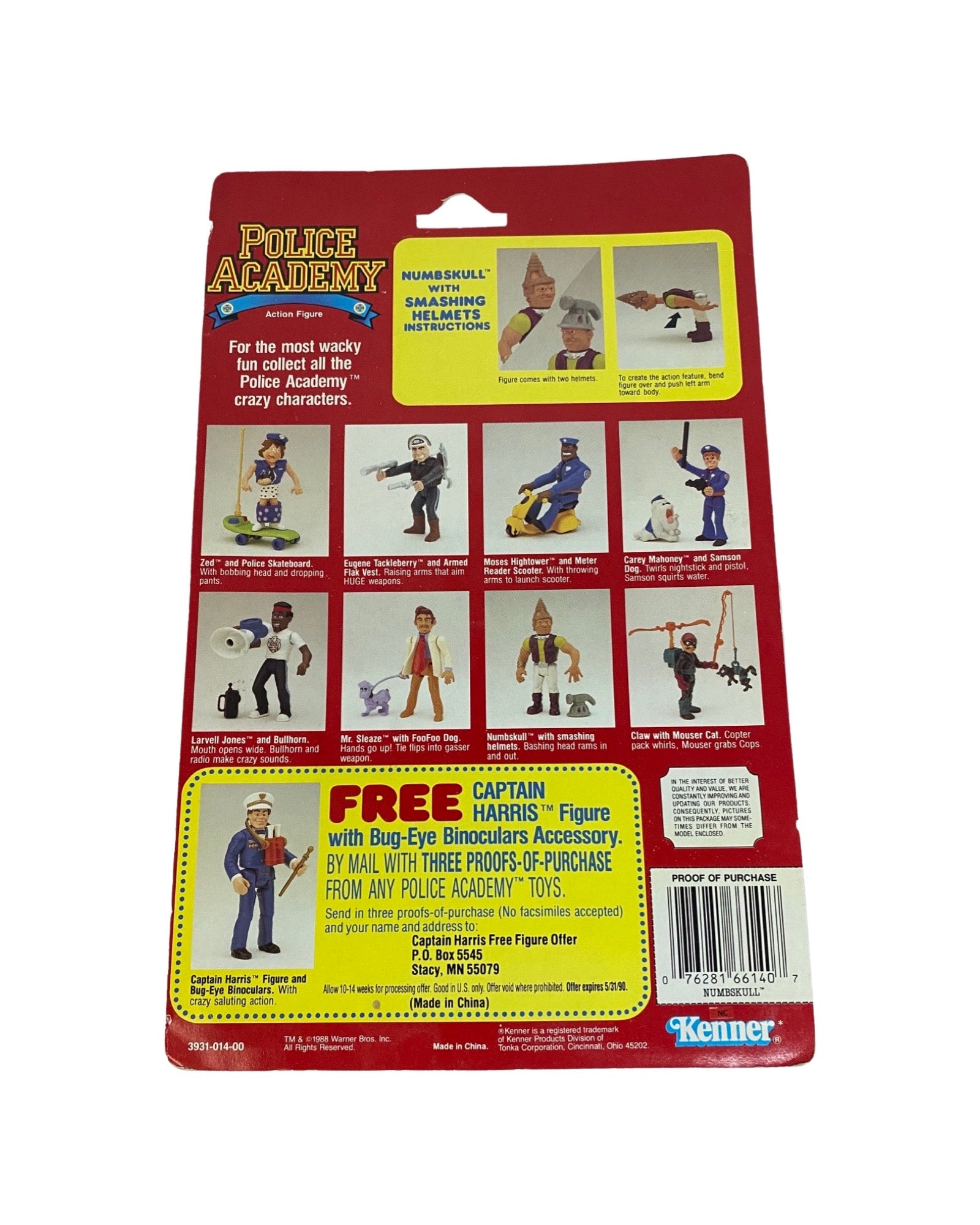This image displays the back of a product package designed for retail, likely meant to hang in a toy store checkout line. The package features a maroon cardboard background and prominently showcases items from Kenner Toys' Police Academy series. At the top left, in large yellow text, it says "Police Academy." Directly below in white text, it reads, "For the most wacky fun, collect all the Police Academy crazy characters." To the right, within a yellow rectangle, the text "Numskull with Smashing Helmets instructions" is highlighted. The package features two rows of four panels, each containing images and descriptions of eight different toy figures and their respective accessories, which include items like guns, a motor scooter, a baton, a loudspeaker, a dog, a pointed hat, and a small manpowered rower flying vehicle. At the bottom, there's a yellow coupon offering a free Captain Harris figure with Bug-Eyed Binoculars accessory by mail, requiring three proofs of purchase from any Police Academy toys. The offer details and mailing address to Captain Harris Free Figure Offer, P.O. Box 5545, Safety, Minnesota 55079, are also provided.